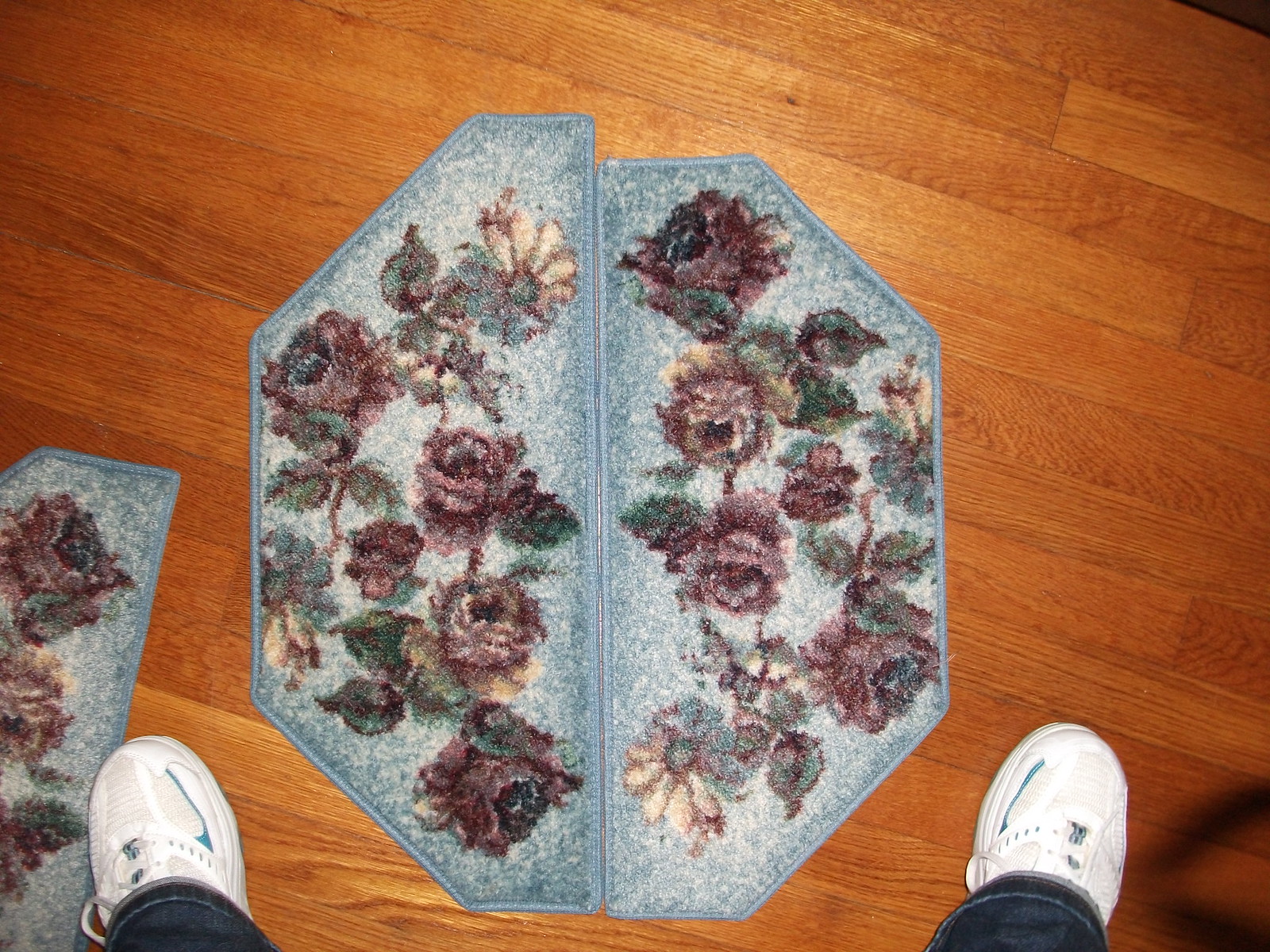This image is a colored photograph taken with a flash, showing a person standing on a beautifully polished light brown hardwood floor. At the bottom of the photograph, you can see the person’s white sneakers – the left sneaker is in the bottom left corner and the right sneaker in the bottom right corner. Part of their jeans cuffs, which appear to be dark gray, are also visible. In the center of the image, there are two pieces of carpet, resembling welcome mats, arranged to form an octagon shape. These rugs have a light blue to slate gray background adorned with dark red roses, maroon flowers that might be daisies or roses, yellow accents, and green leaves. An additional strip of a similar rug design is visible along the right-hand side of the photograph, hinting at a cohesive style. The vertical wooden floorboards beneath them are slightly tilted horizontally from right to left.